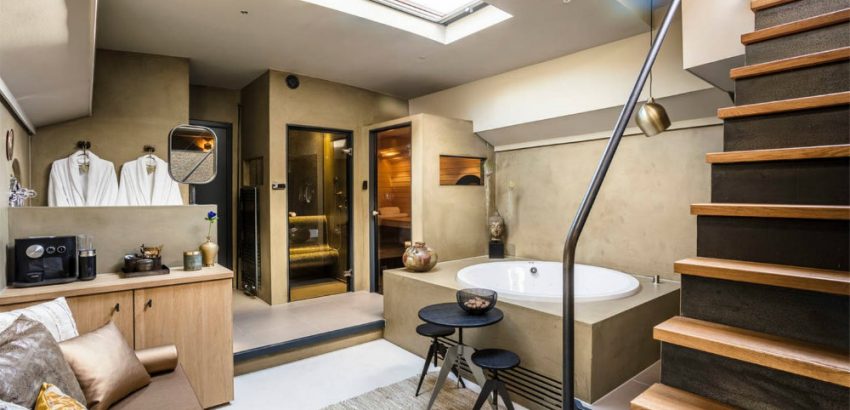This image showcases a luxurious bathroom, possibly in a spa or high-end hotel, featuring an array of elegant and functional elements. To the right, steep wooden stairs descend into the space, flanked by a metal handrail. An inset oval bathtub rests against a wall adorned with brownish-gold hues, complemented by a countertop of the same color. Beside the tub, two pedestal chairs and a small table offer a cozy seating arrangement. Decorative touches include a Buddhist-style ceramic head and a vase placed on the tub's ledge.

In the background, glass-enclosed shower stalls or saunas can be seen, adding to the room's opulent feel. Adjacent to this area, two fuzzy, white robes hang invitingly on hooks next to a square vanity mirror.

The left side of the room features a lounge area with a coppery-gold, rose-gold metallic sofa adorned with pillows. In front of this lounge is a coffee bar, equipped with a coffee maker, cups, and possibly a toaster, all atop cabinets. This detailed and cohesive setup creates a sophisticated and comfortable environment ideal for relaxation and rejuvenation.